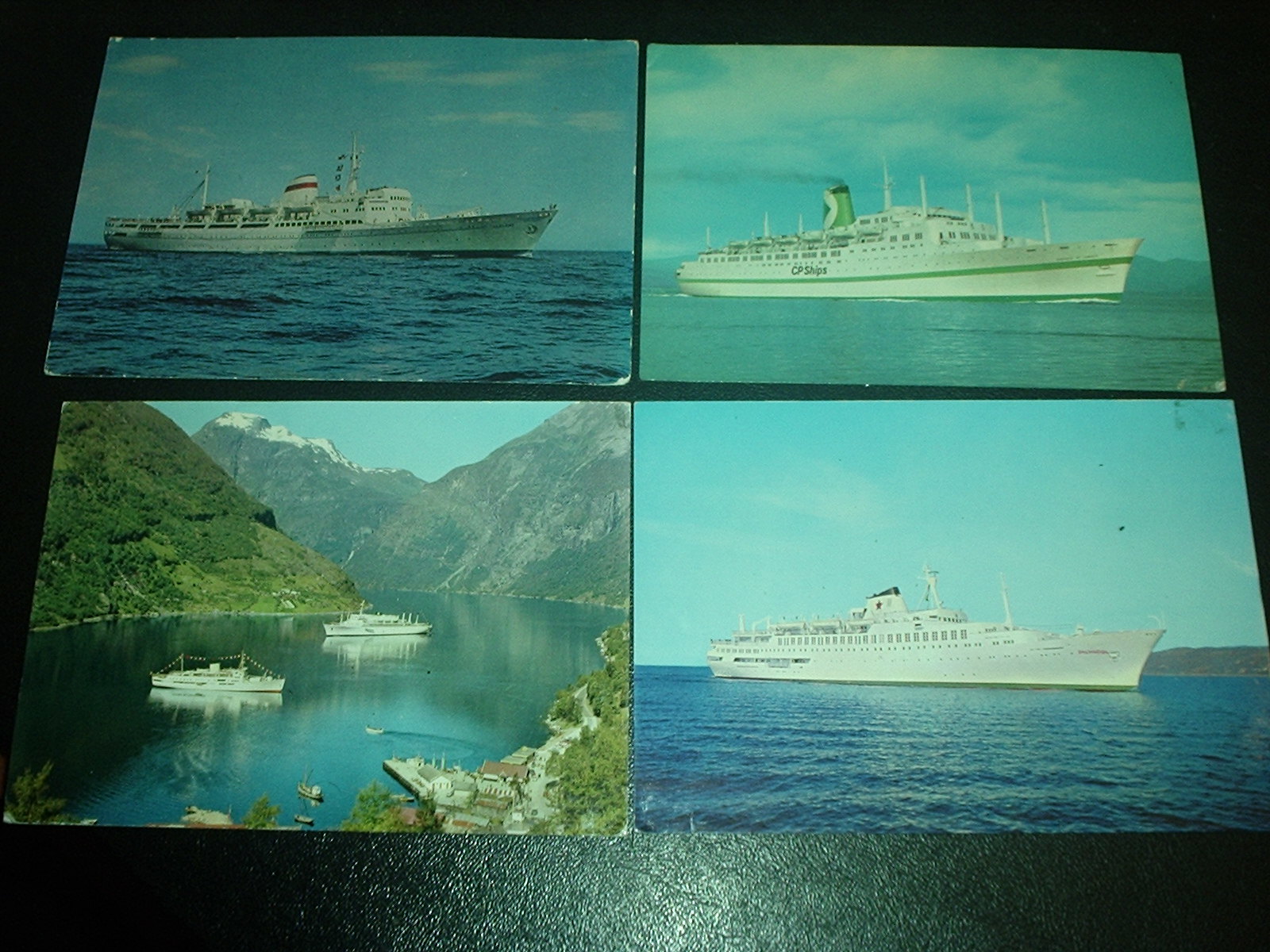This digital photograph captures four smaller, vintage-style photographs arranged in a 2x2 grid, set on a shiny, black vinyl-textured surface. Each smaller photo features white ships, totaling five across all four. The top left photo exhibits a long, white ship set against a dramatic scene of very dark blue water under a sky with bluish and white clouds. To its right, the photo displays a white cruise ship with a distinctive green stripe down the middle of its hull, marked with "O.P. Schiphol" in black font. This ship navigates through less blue, cloudier skies, with a prominent red, white, and blue steam tunnel at the back capped in black. The lower left photograph portrays a river or lake, with two white ships; one in the foreground and one farther back, surrounded by a picturesque landscape featuring a snow-topped brown mountain and a smaller lush green peak with tan and brown rocks and green foliage. The bottom right photo closely resembles the top left, but it includes an additional landmass—a small, brownish hill—on the right side of the picture, enhancing the natural scenery.